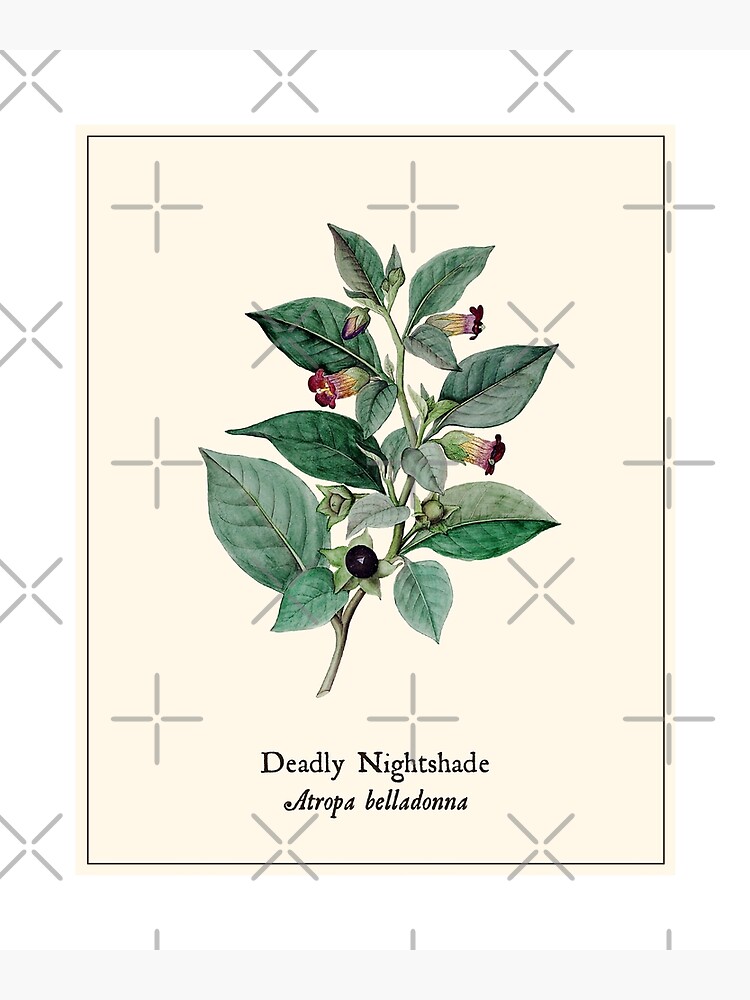This vertically aligned rectangular illustration is framed by a thin black border and set against a beige background. At the center of the image is a short stem sprouting leaves in various shades of dark and medium green, spreading out in all directions. The stem appears to have been cut at an angle at the bottom. Nestled among the leaves are small flowers in various stages of blooming. There are about four or five flowers; one remains a closed, triangular bud, while the other three have begun to open, revealing delicate purple petals.

Across the middle of the image, a watermark reads "larkwort." At the bottom, in centered black text, the image is labeled "deadly nightshade," followed by its scientific name, "atropa belladonna." The plant is depicted with a meticulous attention to detail, emphasizing both the foliage and the partially blooming flowers.